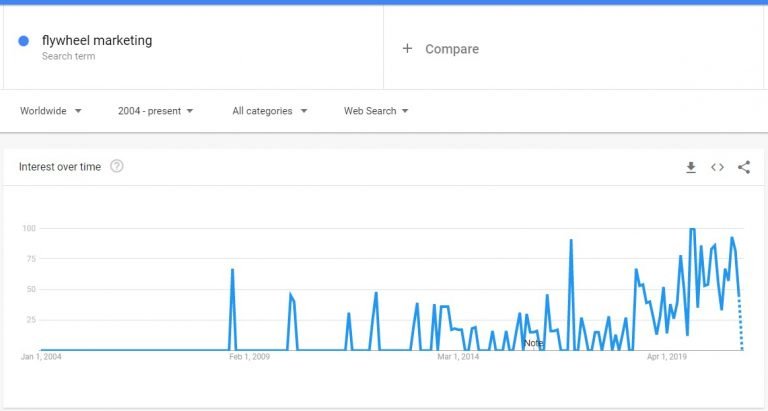This image presents an insightful chart detailing the interest over time of the search term "flywheel marketing" from January 1st, 2004 to the present, encompassing all categories and focusing on web search data worldwide. The timeline is marked with key dates including January 1st, 2004, February 1st, 2009, March 1st, 2014, and April 1st, 2019, allowing for a clear view of trends and patterns. At the top of the chart, a header bar is displayed, colored in shades of blue, black, and white. This visualization aids in understanding the evolving popularity and global reach of "flywheel marketing" over the years.